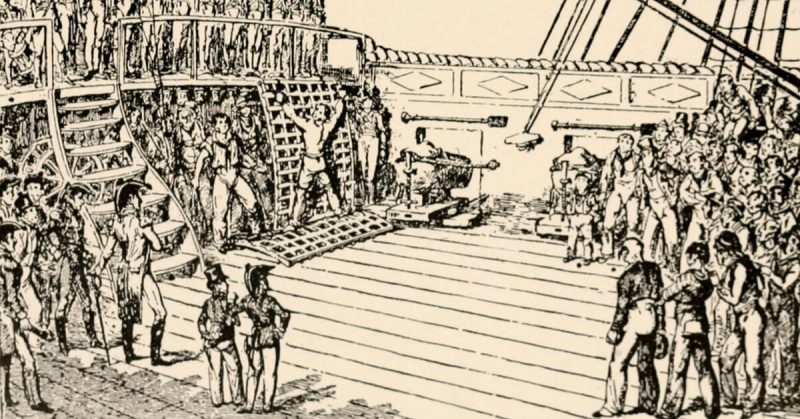The digital screenshot captures a vintage-style, hand-drawn illustration in black ink on yellowed paper, measuring approximately six inches wide by three inches high. Set on the deck of an old wooden ship, likely a Viking or pirate ship, the scene is framed by the deck's long planks, with part of the ship rising to the second level on the left, and rigging lines visible in the upper right-hand corner. 

Centered in the chaotic scene is a man, shirtless and bound spread-eagle to a rack or pallet of wood, positioned slightly left of center. Surrounding him is a large crowd of people, some potentially singing, some brutish, including a man holding a whip, poised to strike as part of a brutal punishment. The ship's crew appears to be dressed as Navy officers, and the right and left sides of the composition are densely populated, creating a stark contrast with the open space around the bound man. This intense, life-at-sea depiction is devoid of any text, drawing the viewer's focus intently to the drama unfolding on the ship's deck.